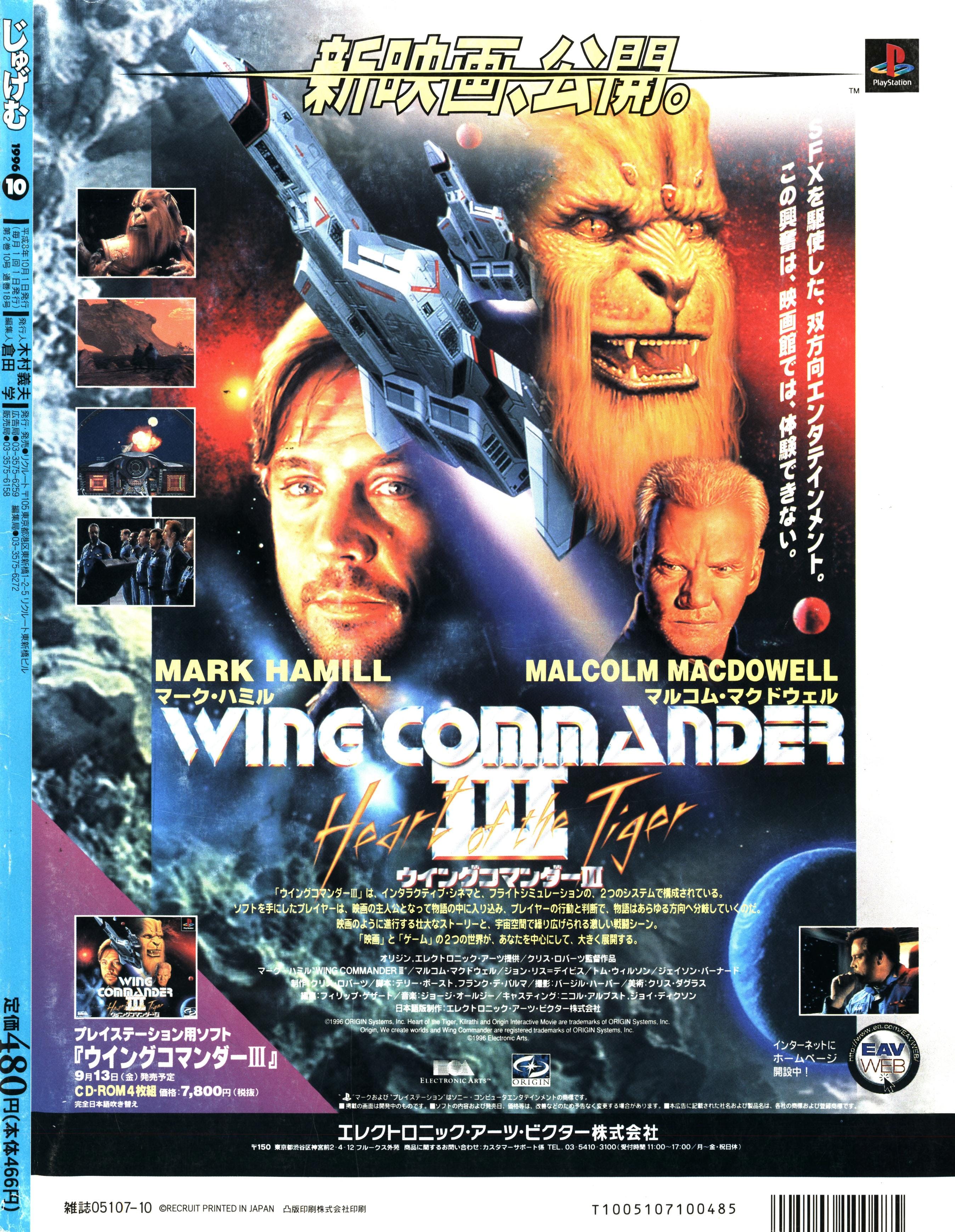This is a vertically oriented Japanese poster for the movie "Wing Commander 3: Heart of the Tiger." Dominating the center-left is a middle-aged Mark Hamill, with his name inscribed below his face. To the center-right is Malcolm McDowell, also labeled with his translated name beneath. At the upper right, a fierce, lion-like creature gazes outward, adding an element of intrigue. Between the two main actors, a spaceship soars toward the top left, highlighting the film's sci-fi theme. Four smaller image squares run down the left side, portraying various scenes from the movie. The title "Wing Commander 3: Heart of the Tiger" stretches visibly across the bottom, accompanied by additional Japanese text. Below, there's a collection of characters, including the number 480, and a barcode. The color palette ranges from orange, beige, tan, gray, white, blue, red, to black, enhancing the overall dynamic look of the poster.